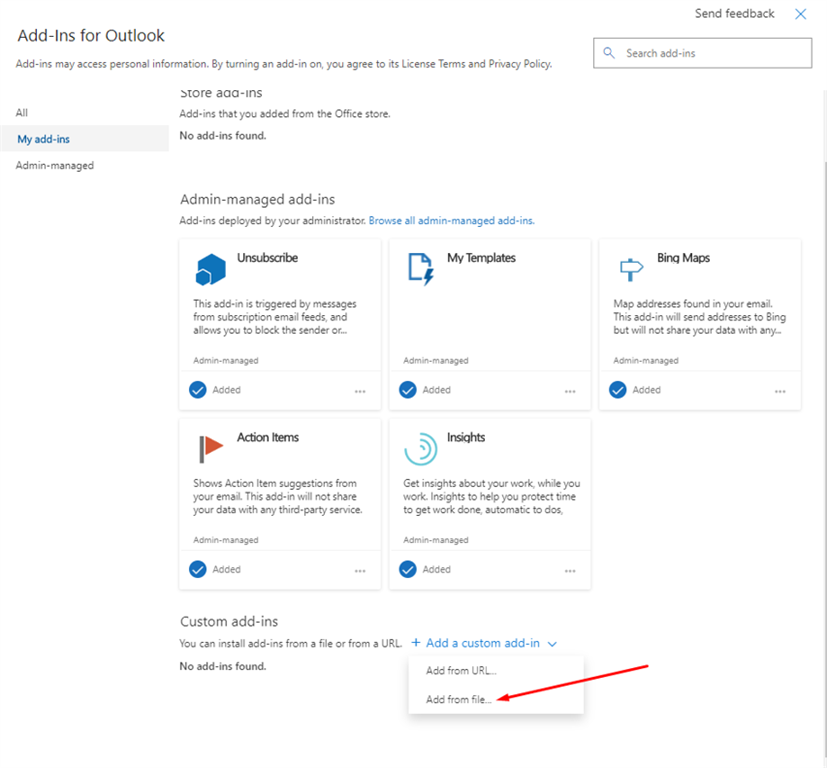This image displays a computer screen showcasing the "My Add-Ins" page for Outlook. At the very top left, the title "Add-ins for Outlook" is prominently written in bold black text. Just below, a sentence in black states, "Add-ins may access personal information. By turning an add-in on, you agree to the license terms and privacy policy." 

In the top right corner of the screen, "Send feedback" is written with a blue 'X' symbol next to it. Below this, there is a search bar for easy navigation. To the left, there are three categories listed: "All," "My Add-ins," and "Admin-managed." The "My Add-ins" category is currently selected.

Adjacent to this, "Admin-managed add-ins" is displayed. There are five add-in categories listed: "Unsubscribe," "My Templates," "Bing Maps," "Action Items," and "Insights." Each category (except "My Templates") includes a brief description in black text. Notably, "My Templates" has no text description, only the label "Admin managed." All five categories have a blue check mark indicating they are "Added."

Towards the bottom of the page, the section titled "Custom Add-ins" provides options to install add-ins from a file or a URL. To the right of this is a blue link labeled "Add a custom add-in," with dropdown options to either "Add from URL" or "Add from a file." A prominent red arrow points directly at the "Add from file" option. The entire interface is set against a clean, white background.